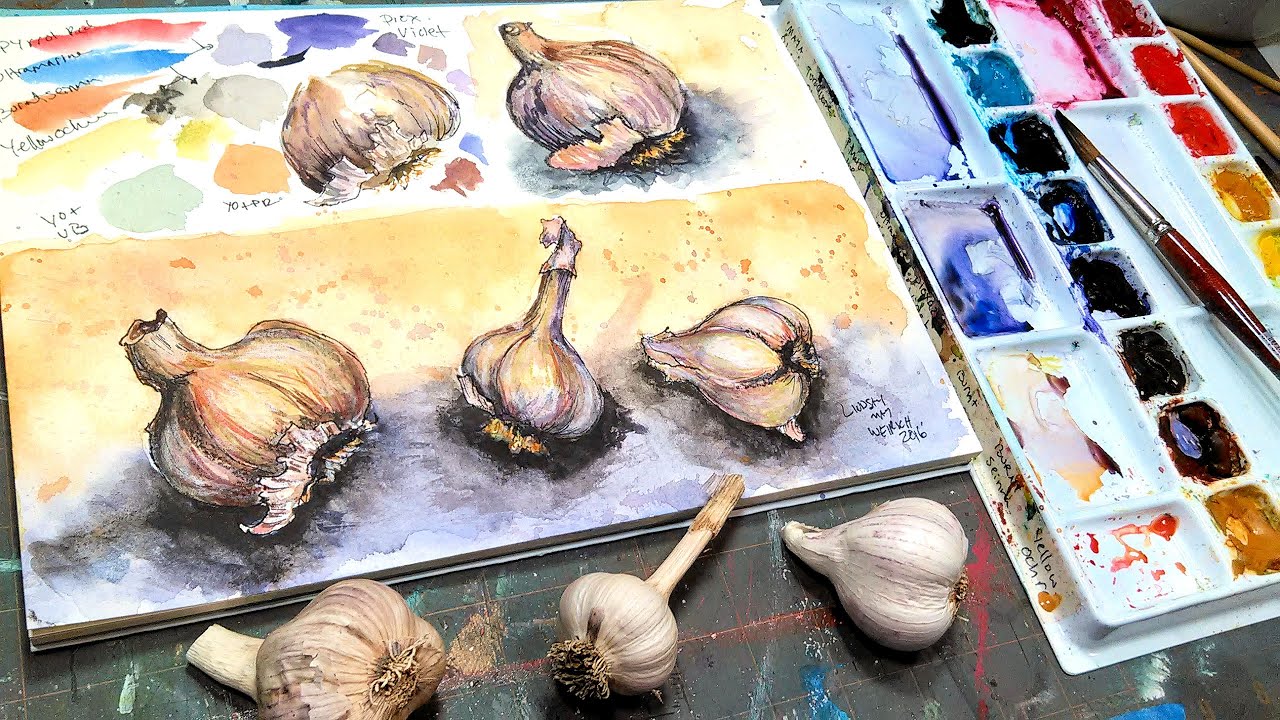This image captures an artist's workspace from a top angle, showcasing a watercolor painting in progress. In the foreground, three identical garlic bulbs are used as models. The painting features these bulbs, brought to life in shades of yellow and brown, resting on a pale gray surface with a subtle yellow background. To the right of the canvas lies a tray of watercolor paints in various hues—dark blue, yellow, red, pink, and purple—with a paintbrush balanced across the middle. The workspace is set on a large green table, which also holds other items of interest such as unfinished sketches of garlic cloves and color swabs, including handwritten notes. Indistinguishable writing is present in the lower right-hand corner of the painting, alongside the artist's name, Lindsay, and the date, 2016. The composition captures the meticulous process and vibrant palette of the artist at work.